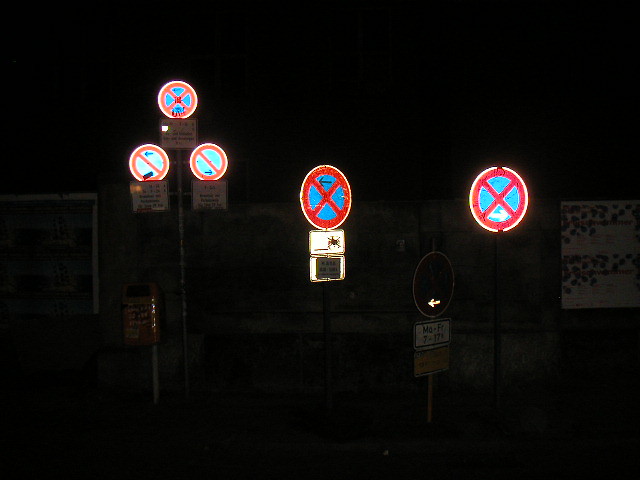This color photograph depicts a very dark night scene with a nearly indistinguishable ground and a completely black sky. The only visible elements are several illuminated round road signs mounted on steel poles. Towards the upper left corner, three signs are positioned almost on top of each other in a triangular formation on the same pole. The top sign features a red circle with a red X dividing it into four blue segments. The two signs below it, placed side by side, each show a red circle with a diagonal red line across a blue background. All three of these signs have small white square panels with text underneath them, although the text is not legible in the photograph. In the middle of the image, there is a solitary sign with a red circle and a red X through a blue background, also having a small white box beneath it. On the far right, two more signs with the red X and blue background are visible, again accompanied by a small white box at the base of one. Additionally, there appears to be a larger, squarish, nearly rectangular object with possible ink splotches near the right-hand edge of the image. Several dimly lit, indistinguishable objects populate the rest of the almost black background.